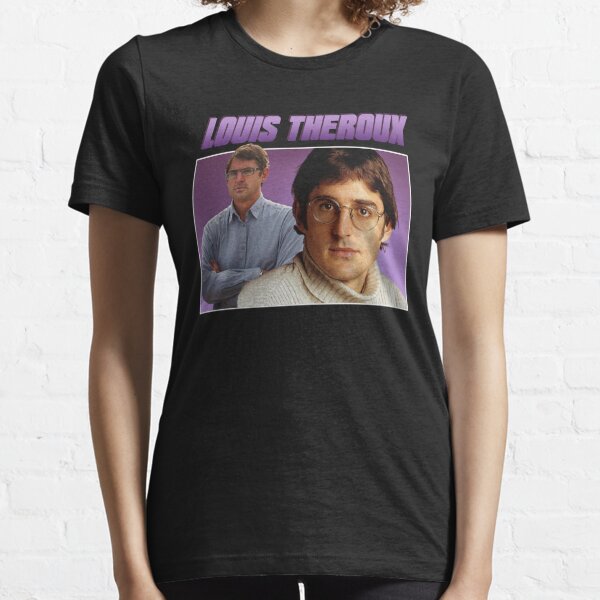The image features a slim, slender woman modeling a black, short-sleeved cotton t-shirt. Her face is cropped out of the frame, but her curly brown hair is visible, along with her neck and arms, which rest akimbo. She seems to be wearing black pants, though they are mostly obscured. The focal point is the graphic on the t-shirt, displaying the name "Louis Thoreau" in bold, uppercase purple text. Central to the shirt are two photos of Louis Thoreau within a purple square with a white border. In the right photo, Thoreau's face is shown close-up, wearing glasses and a white woolen turtleneck. The left image captures him from the waist up in a blue button-up shirt, also with an intense expression and glasses. The model stands against a white brick wall, drawing all attention to the detailed design of the t-shirt.